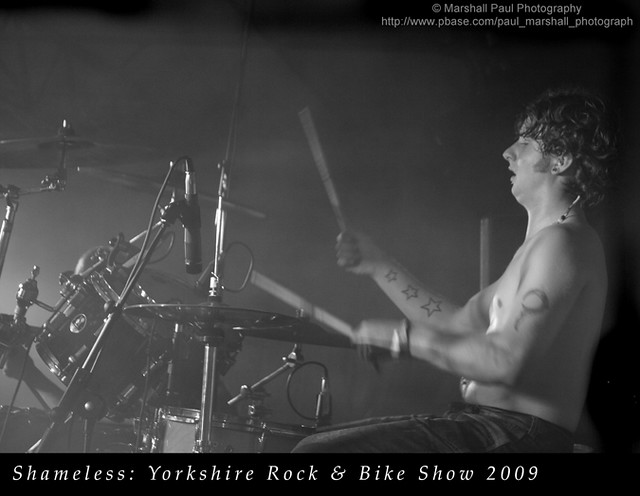This is a black and white photograph capturing a shirtless drummer live on stage. The drummer, positioned on the right, has long, shaggy brown hair and sideburns reaching his earlobes, both drenched in sweat. He is seen in profile, mid-performance, with drumsticks in hand, simultaneously striking cymbals and tom-toms. His right forearm features a tattoo with three stars of increasing size, and there appears to be another tattoo on his left bicep. In front of him, a full drum set and a microphone stand are visible against a black and gray backdrop. Detailed text overlays the image: the top right corner reads "Marshall Paul Photography" followed by a URL (http://www.pbase.com/Paul_Marshall_photograph), while the bottom contains a black bar with the white text "Shameless: Yorkshire Rock and Bike Show, 2009." The photograph exudes a raw, energetic intensity, emblematic of a high-energy performance.